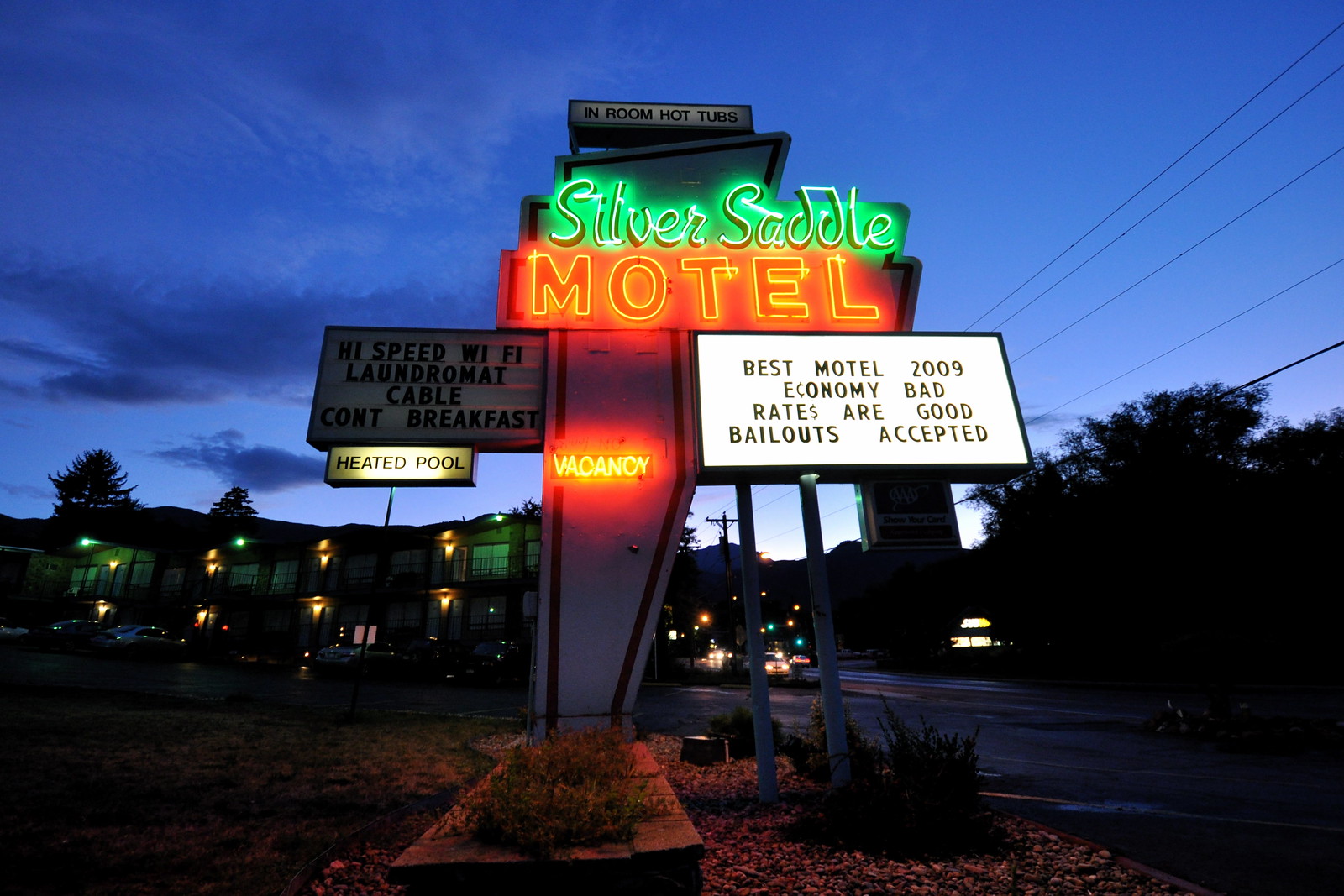The image depicts an outdoor setting during dusk or dawn, showcasing a prominent neon sign towering 20 to 30 feet high. Central to the scene, the sign reads "Silver Saddle Motel" in green and red neon lights, respectively. Below this, another neon sign spells out "Vacancy" in orange-yellow letters. Adjacent to these, a white sign displays in black print: "Best Motel 2009, Economy Bad, Rates Are Good, Bailouts Accepted." Off to the right, an additional white neon sign indicates "Heated Pool" in black neon lettering.

Surrounding the sign, the landscape includes a grassy ground surface, a roadway to the right, and various trees. In the background, a two-story motel building is visible, illuminated by exterior lights. The sky above transitions from a lighter to a darker blue, indicating the time of day. The colors in the image span blue, green, red, orange, yellow, black, gray, and brown, enhancing the vividness of the scene.